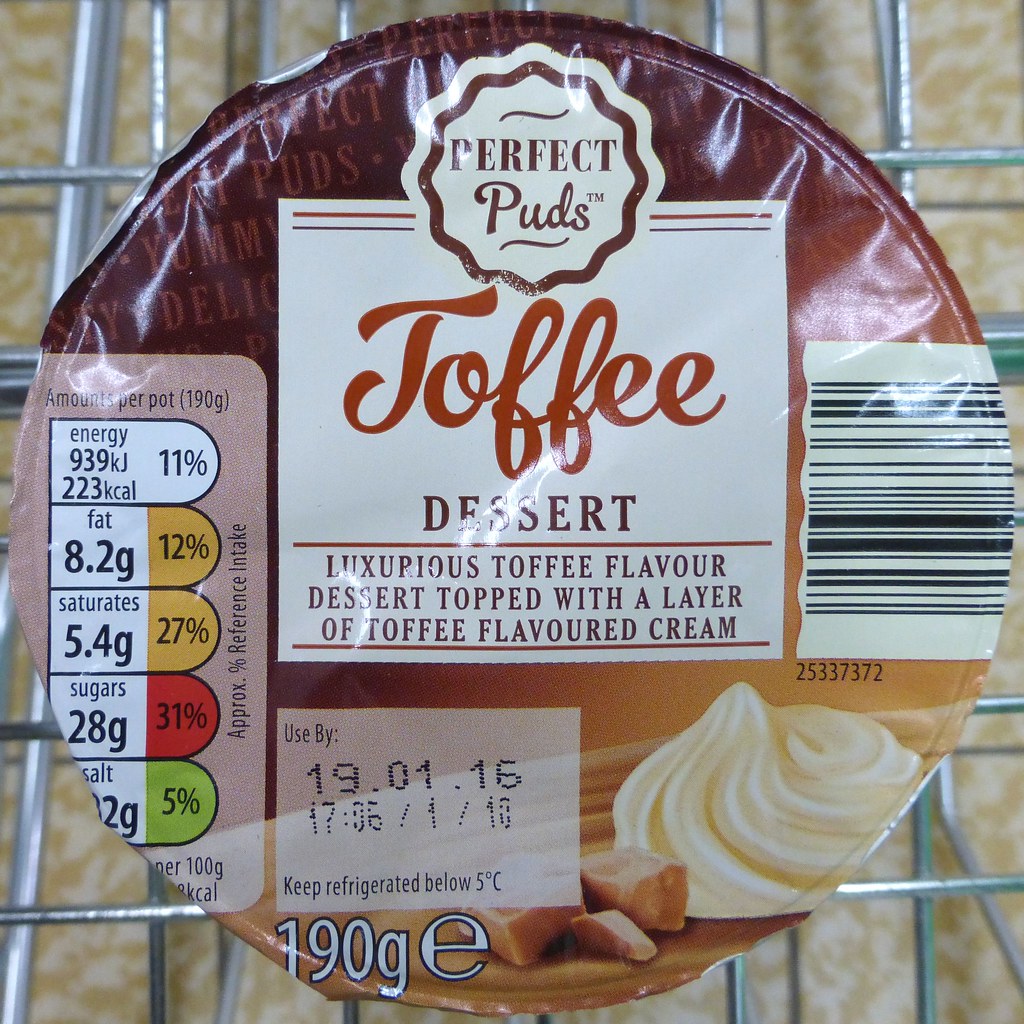This color photograph features a close-up, top-down view of a circular package for a toffee-flavored dessert. The background of the image consists of crisscross metal bars or a wire rack atop tan and white cloud-patterned tiles. The package design is split with a brown upper section and a tan lower section. 

On the top of the circle is a logo within a scalloped border, containing the words "PERFECT PUDS" and a "TM" mark. Directly below, a white rectangular panel showcases the word "TOFFEE" in prominent brown cursive, and underneath, "DESSERT" in bold caps, followed by the phrase "LUXURIOUS TOFFEE FLAVOR DESSERT topped with a layer of toffee-flavored cream" in Times New Roman. Off to the right side, a barcode with the sequence "25337372" is present.

To the left of the package, a pink background encloses a vertically aligned rectangular nutrition information panel. Here, horizontally aligned bullet shapes detail the nutritional facts: "NRG 939KJ" and "23KCAL" at the top, followed by "Fat 8.2g" in yellow, "Saturates 5.4g" in yellow, "Sugars 28g" in red, and "Salt 2g" in green, each with their respective percentage values (11%, 12%, 27%, 31%, 5%). Below the bullets, the text “100g” and “approximate reference intake” is displayed. 

A pink horizontal rectangle on the upper-left side documents the use-by date as "19.1.16," with further details "17.6.1.10" and a storage instruction to “keep refrigerated below 5C.” Just below this, in white text, the package weight "190g" is noted next to a lowercase "e."

Visual elements include pieces of presumably toffee on the right and a dollop of whipped cream or meringue, reinforcing the luxurious and creamy nature of the dessert. The entire composition and layout leverage a photographic representationalism style, typical of product photography aimed at highlighting the dessert's indulgent appeal.